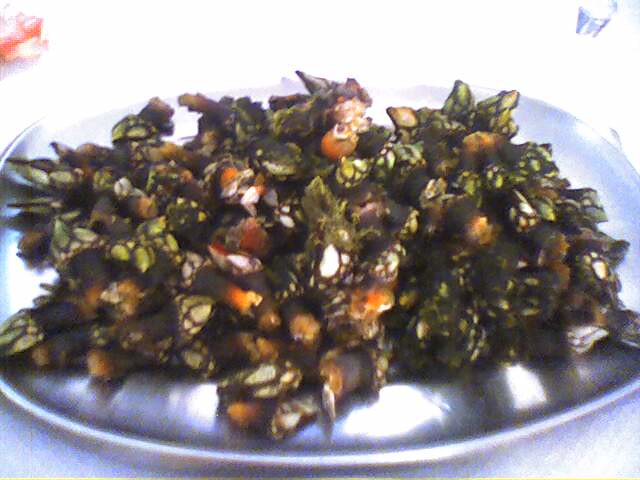The photograph captures a meal, likely taken in a restaurant, featuring a somewhat blurry image of a silver plate on a blindingly bright white tablecloth. The dish appears to be a vegetable-based item, resembling asparagus, interspersed with bulbous elements and possibly charred or burnt areas that show shades of brown and black. The predominantly green asparagus also features hints of orange. The food is spread in a single layer, nearly covering the entire plate, with only the edges of the silver plate visible. In the background, towards the top right, there's the faint outline of a glass, and to the top left, a light red object can be discerned, though much of the finer details are obscured by a harsh flash of light, making the overall image difficult to describe with precision. The reflection on the plate suggests that the setting is indoors, likely lit by strong overhead lights.